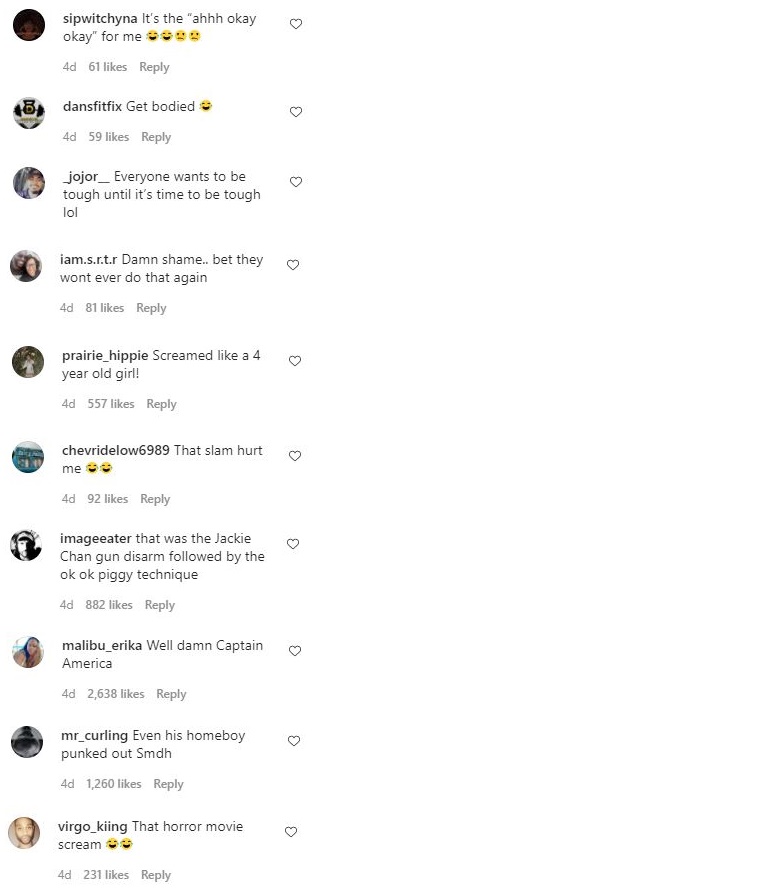The image showcases a detailed comment section from a social media post. There are a total of ten comments displayed, each accompanied by corresponding user profiles, heart icons to like the comments, like buttons, reply buttons, and timestamps indicating when each comment was posted. 

The top comment is from a user named Sip Wichina, stating, "it's the, ah, OK, OK for me." Directly underneath, another user named Dan's Fit Fix comments, "get bodied."

Uniquely, there is one prominent post from the user JOJR, saying, "Everyone wants to be tough until it's time to be tough, LOL." This comment is distinctively highlighted as it lacks a timestamp, like, and reply options, but it does feature a heart icon next to it. This suggests it might be a featured or pinned comment.